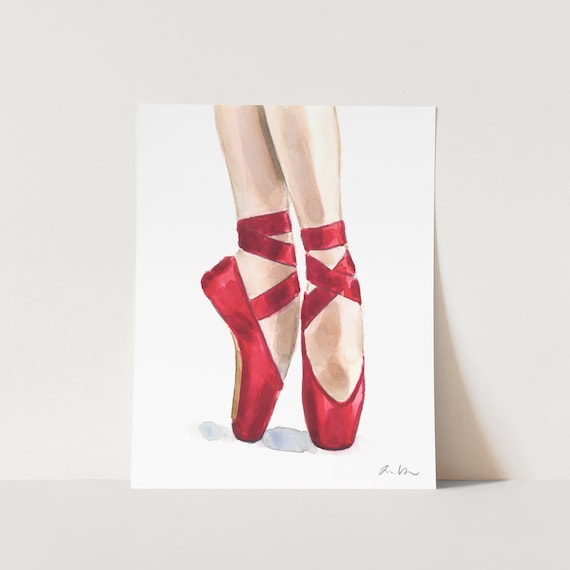This detailed artwork captures a close-up of a ballet dancer's lower legs and feet, meticulously painted against a subtle, creamy white background. The focal point is the dancer's feet adorned in shiny red ballet shoes, with thick red straps crisscrossing and looping around her tiny ankles. One foot is elegantly positioned on its very tiptoe, showing the flat-front design typical of pointe shoes, while the other foot is turned to the side, arching gracefully. The soles of the shoes are brown, contrasting with the pristine white of her tights, and a soft shadow subtly extends from her feet onto the white paper below. The painting is signed in cursive at the bottom right corner, adding an authentic touch to this exquisite artistic depiction.